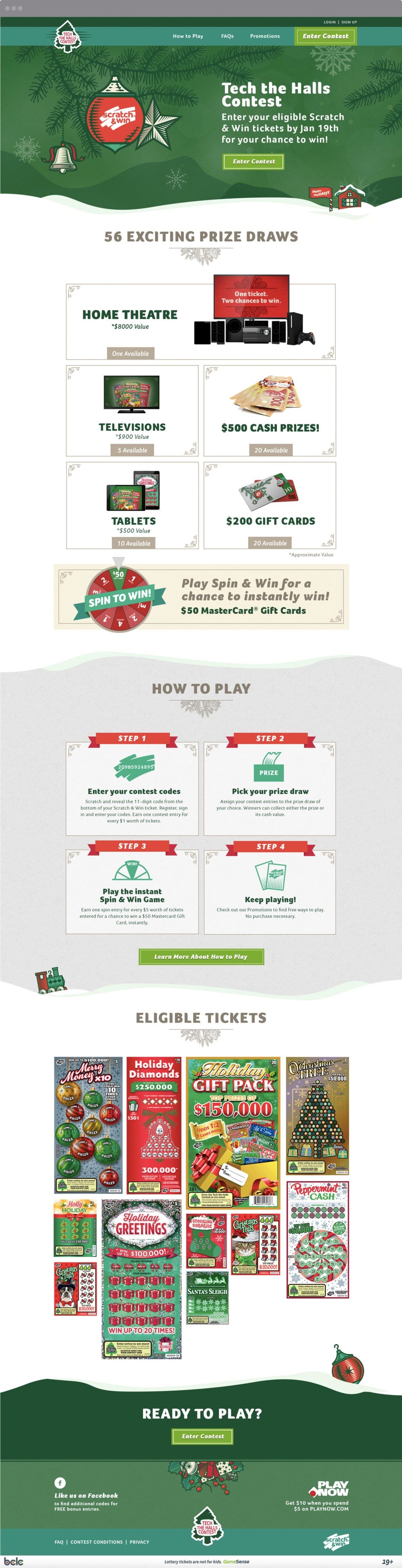"Detailed promotional flyer for the 'Tech the Halls' contest: This small but intriguing flyer announces the 'Tech the Halls' contest, featuring a total of 56 exciting prize draws. Central to these draws is a grand prize that includes a complete home theater system. Additional prizes include state-of-the-art televisions, $500 cash awards, tablets, and $200 gift cards. Furthermore, participants have the chance to instantly win $50 MasterCard gift cards by playing the 'Spin and Win' game.

The flyer outlines how to participate in four steps, though the text is too small to discern clearly. It mentions that the contest is accessible through eligible lottery tickets, implying a second-chance promotion for non-winning tickets. The eligible tickets are presented as a numbered list, showcasing nine different ways to enter. This promotional flyer seems to be part of a larger online initiative, encouraging players who have lost in the lottery to enter for a chance to win various tech prizes."